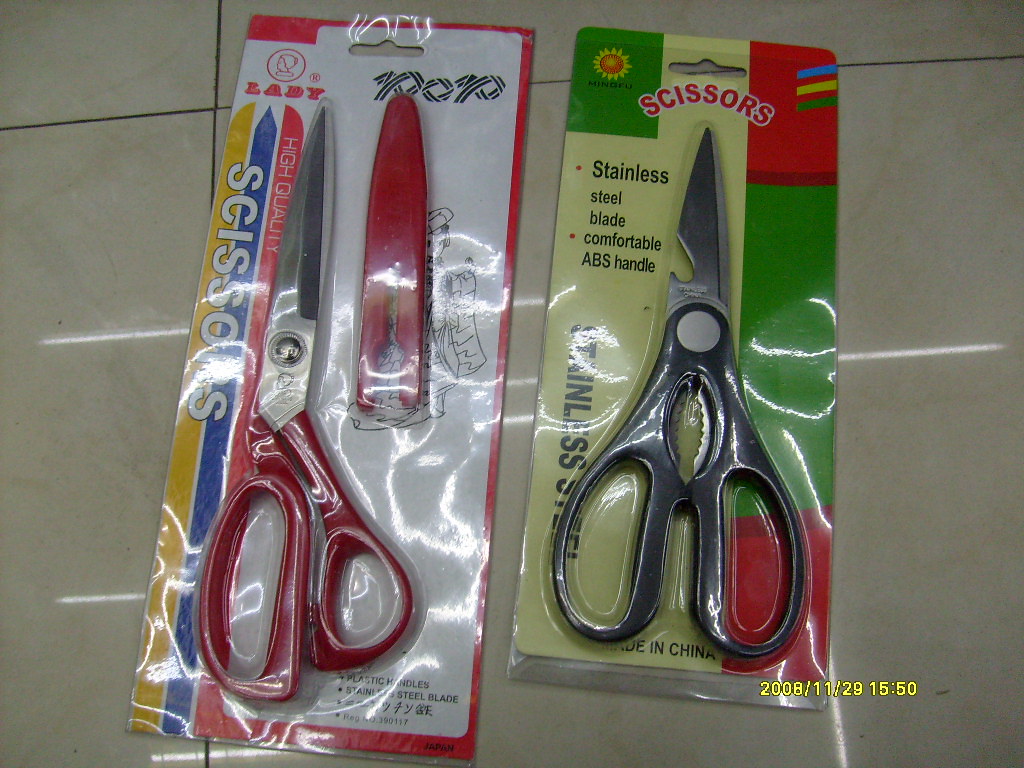This image, timestamped 2008-11-29, 15:50 in yellow text at the bottom right, features two pairs of scissors in their unopened packaging, placed side-by-side on a beige tiled floor with dark grout lines. The scissors on the right are housed in a red, green, and yellow package with text including "scissors," "stainless steel blade," and "comfortable ABS handle." These black-handled scissors, made in China, are described as stainless steel with a distinctive metal area between the handles, possibly for bottle opening, and a shorter blade secured with a round screw. The left pair of scissors, encased in a white package with a red border and protective red blade cover, boasts a red plastic handle and stainless steel blade. The package highlights "high quality" and features a colorful design with stripes of yellow, blue, and red, overlaying which is the word "scissors" in white letters.